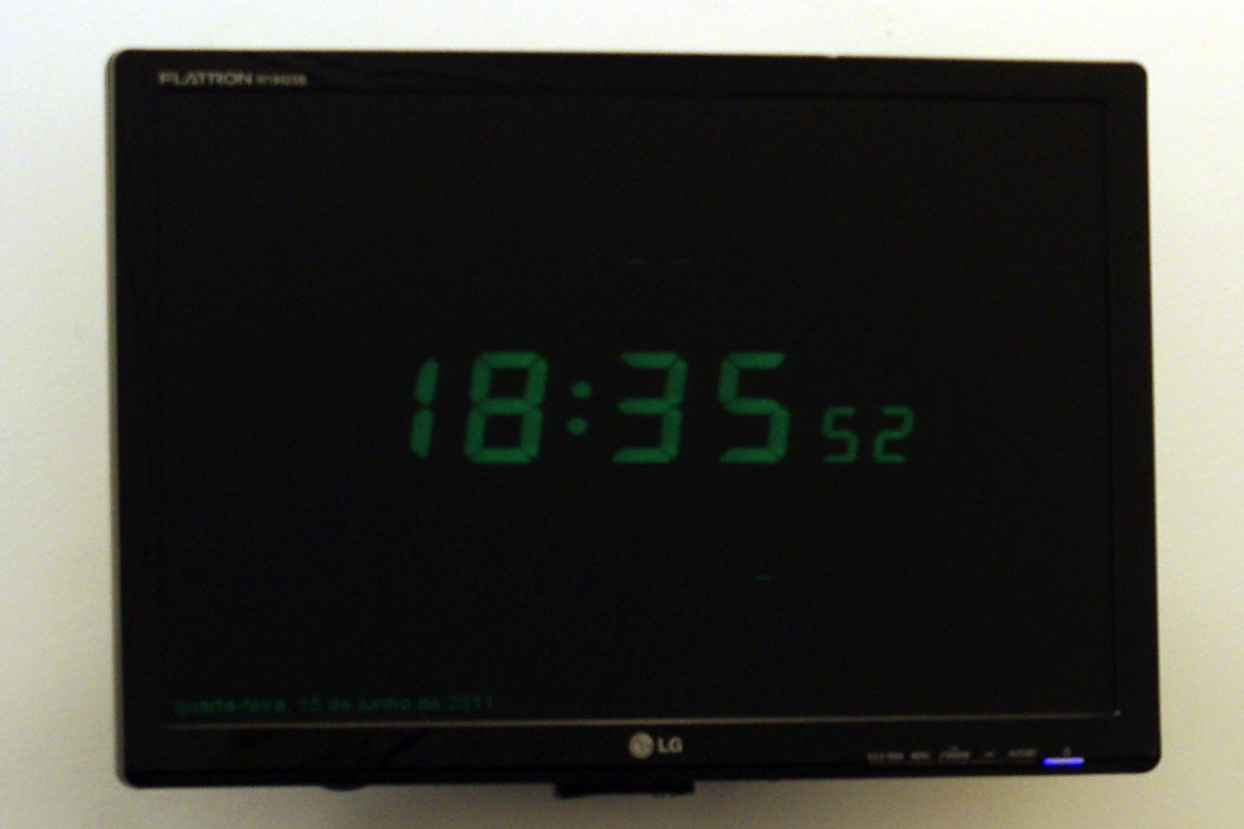The image showcases a flat screen mounted on a white wall, which could either be a television or a monitoring screen. The screen is framed with a black border. In the upper left corner of the border, the word "FLATRON" is prominently displayed, followed by a string of indistinct digits. The bottom middle of the screen features the LG logo. In the bottom right corner, there are purple dotted lights accompanied by small white print, which is illegible. The screen itself displays the time "18:35" alongside a smaller number "52," both rendered in a bright green color.